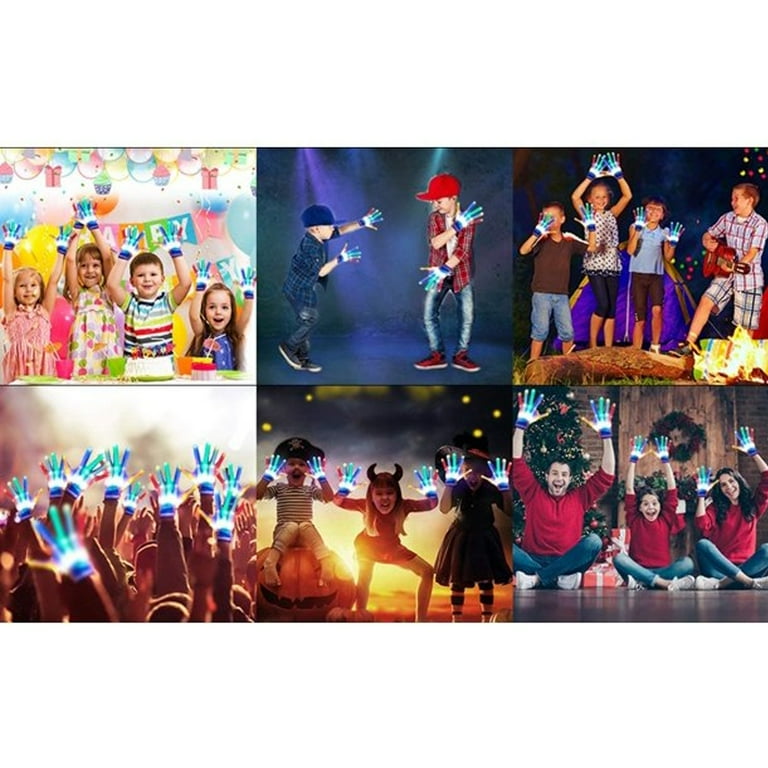This horizontally aligned rectangular image is comprised of six smaller square photographs, organized in two rows of three. Each photograph features children prominently, many of whom are wearing white gloves with brightly colored fingers. The top left picture captures a vibrant birthday party scene with four children enthusiastically raising their hands, against a backdrop of a colorful "Happy Birthday" banner and a cake. In the top center, two boys dressed in blue and red flannel shirts with matching caps perform dance moves, their hands gloved and fingers vividly colored. Moving to the top right, a trio of children dance with their hands up while another child plays a guitar. The bottom row starts with several people seen from behind, their glowing hands raised as if at a concert. The bottom center showcases three children in festive Halloween costumes—a pirate, a devil, and possibly a witch—each displaying their colorful gloves. Finally, the bottom right features a family—an older man, a child in the center, and an older woman—all seated with their hands held high, revealing the same distinct gloves with multi-colored fingers.